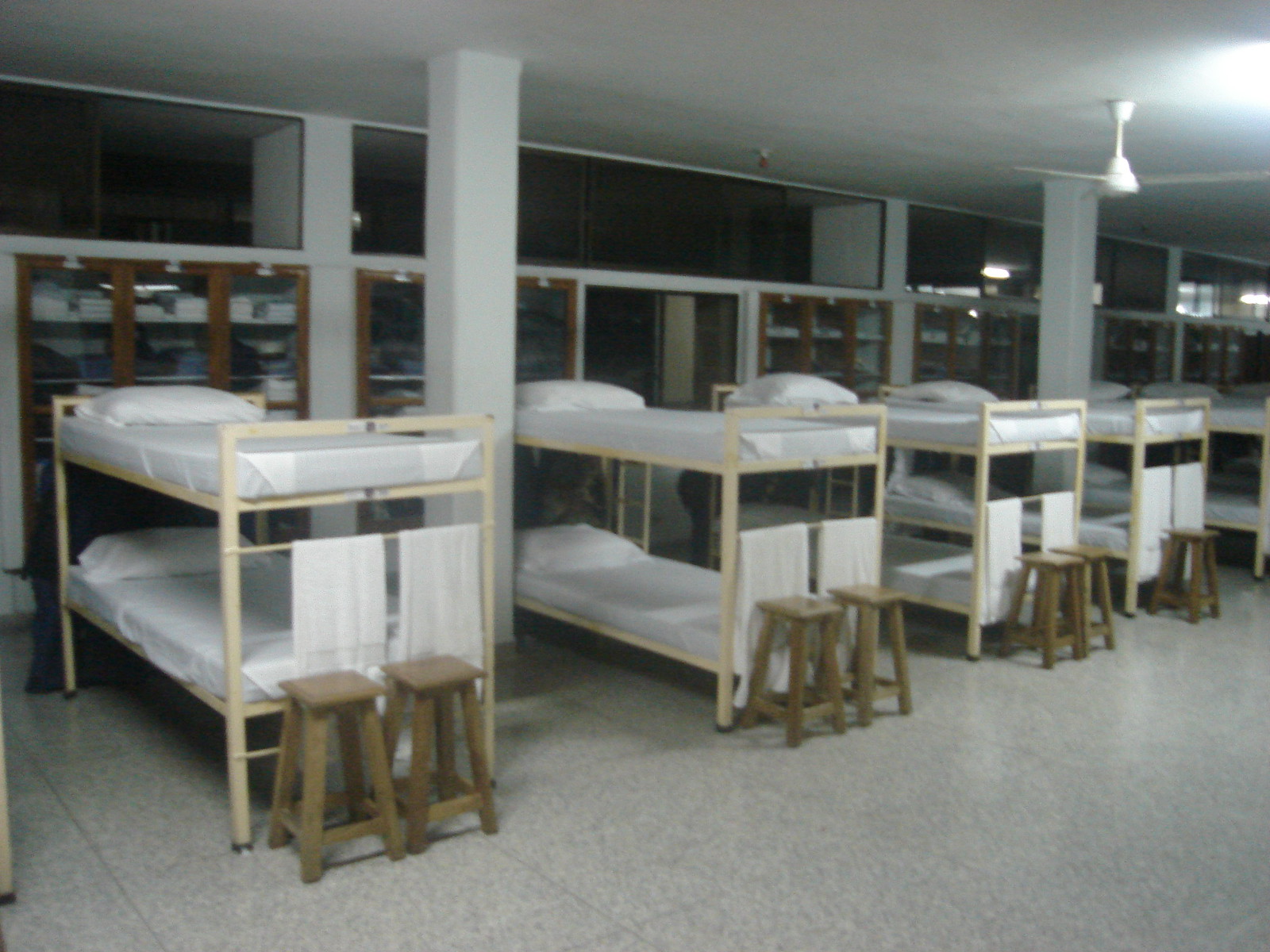The photograph depicts an indoor dormitory setting, which could be from a university, prison, or military barracks. The space features at least five metal-framed bunk beds with a cream color, each equipped with white linens, a flat white pillow, and a pair of white towels hanging from the upper bunks. In front of every bunk bed are two wooden square stools. The dormitory also contains white ceiling support beams and a shiny, gray linoleum floor. Along one wall, windowed doors framed with darker wood are visible, adding contrast to the space. Additionally, a white ceiling fan is installed, contributing to the utilitarian feel of the room. Rows of cubby holes extend horizontally from one end of the photo to the other, providing storage for personal belongings.